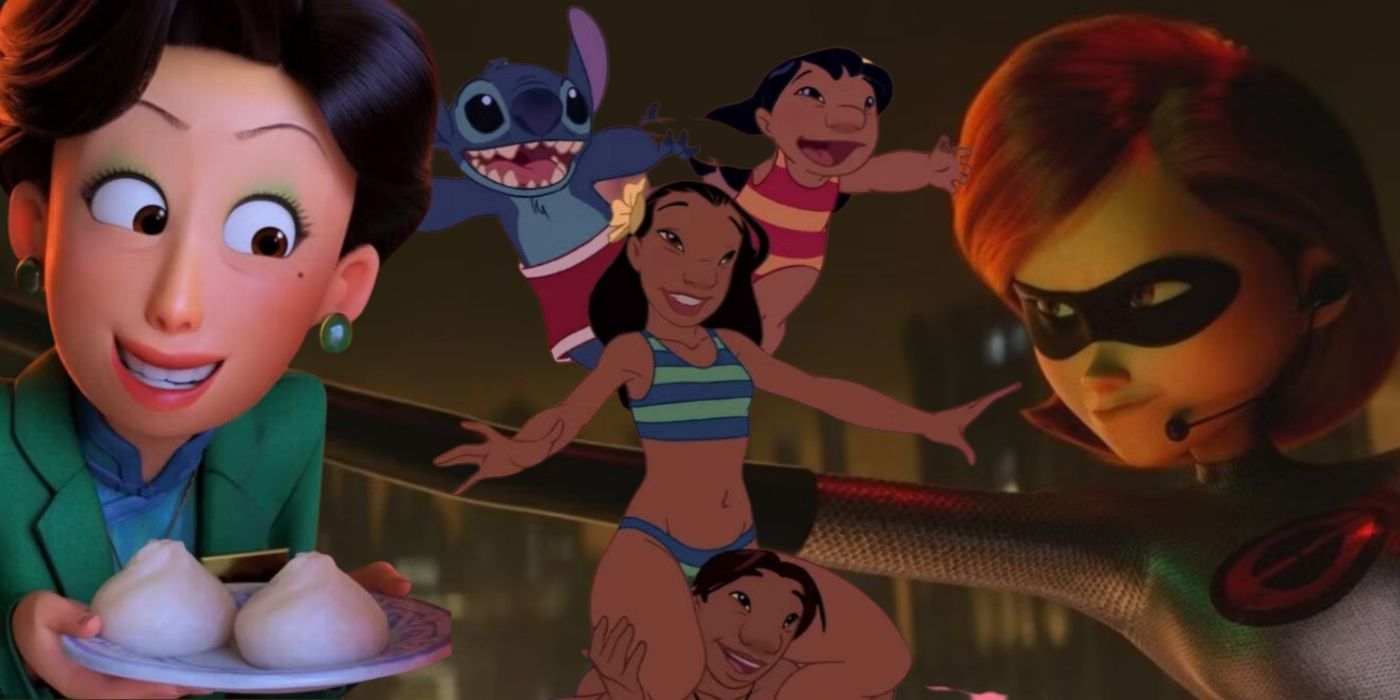This image features a collage of characters from various Disney movies. On the right, a still from "The Incredibles" showcases Elastigirl, the mother with red bob-like hair, a black mask over her eyes, and a silvery suit with a red logo on the front. She is stretching her arm out towards the left side of the image. To the left, in the middle section, we see characters from the movie "Lilo and Stitch." A girl in a red and yellow swimsuit sits atop a guy’s shoulders, and beside her is Stitch, the blue alien with big blue eyes and oversized ears. On the far left, a character from "Turning Red," likely the mother, is depicted with smiling eyes, black hair, and dressed in an aquamarine suit with a blue top underneath. She is holding a plate with two buns, seemingly offering them forward. The overall composition combines these three distinct animations into a single, detailed panorama.